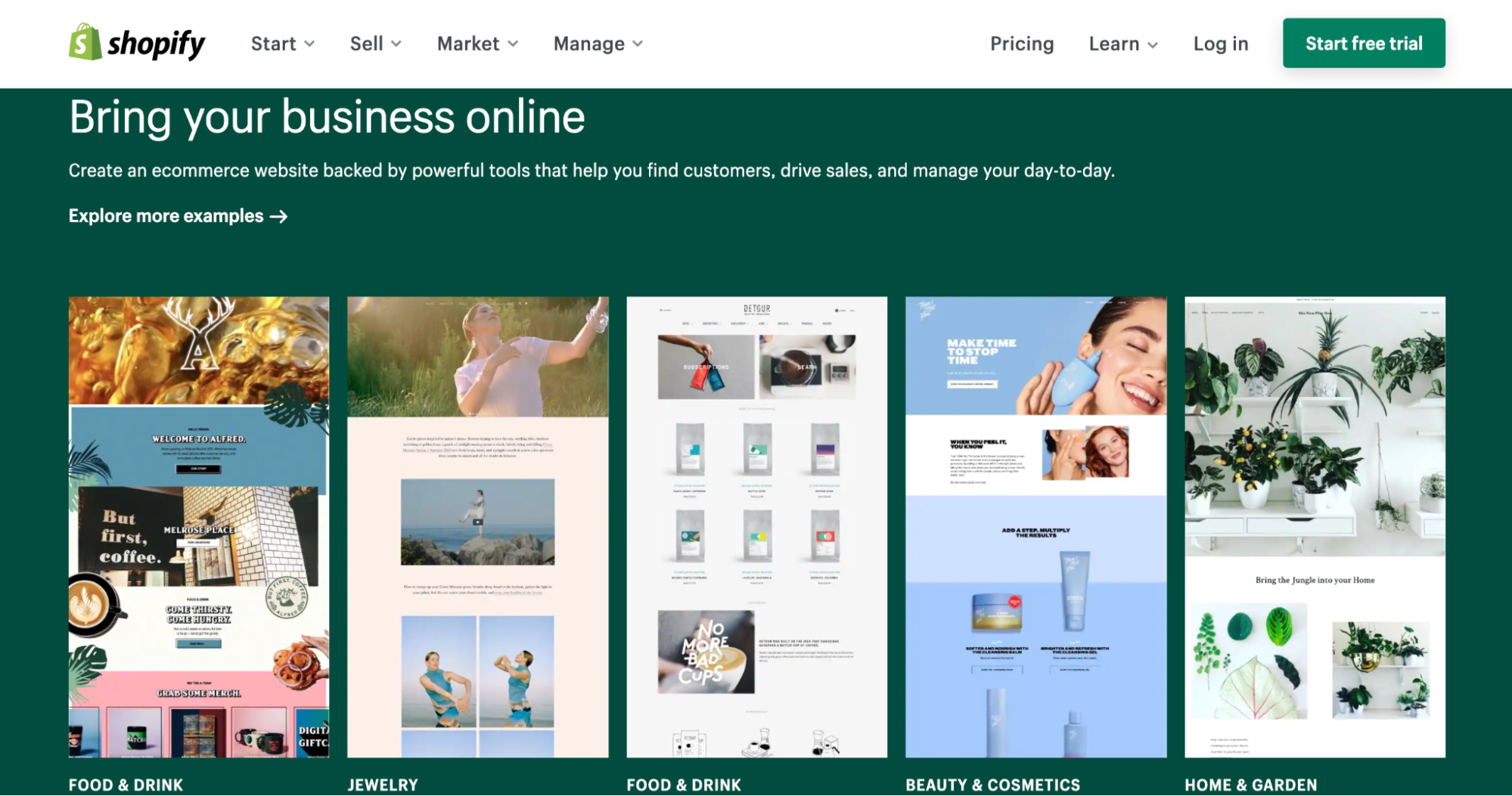In this detailed screenshot of a Shopify webpage, the layout begins with the Shopify logo on the far left—a green shopping bag featuring a white "S". Next to the logo is the word "Shopify" in black italicized font. To the right of the logo, several gray drop-down items are listed: "Start," "Sell," "Market," and "Manage."

Moving further to the right, the navigation options include "Pricing," a drop-down menu labeled "Learn," and a "Login" button. Adjacent to these is a prominent green button, slightly lighter than a Christmas tree green, with white font that reads "Start free trial."

The page features an evergreen-colored background with white text stating "Bring your business online." Below this, in smaller white font, it says, "Create an e-commerce website backed by powerful tools that help you find customers, drive sales, and manage your day-to-day." In bold white text, it then prompts, "Explore more examples."

To provide users with starting points for their Shopify site, the page showcases various example templates including a "Food and Drink" template, a "Jewelry" template, another "Food and Drink" template, a "Beauty and Cosmetics" template, and a "Home and Garden" template.